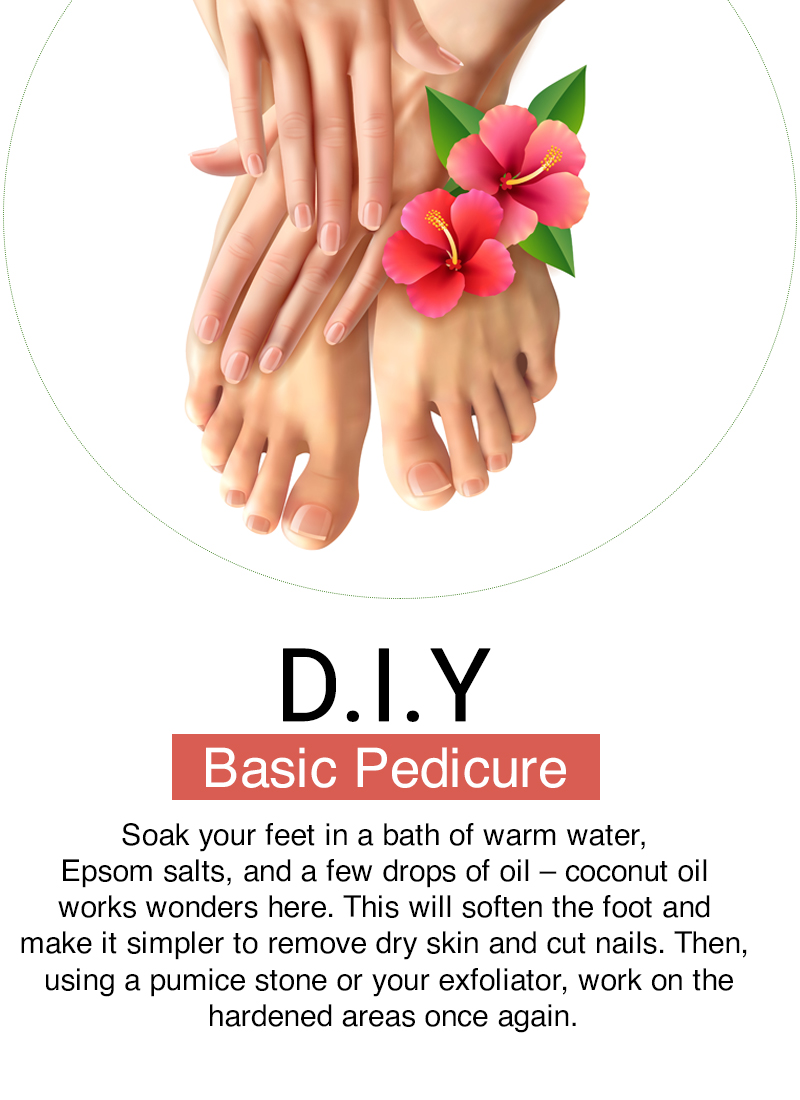The image is an educational illustration on how to perform a basic do-it-yourself pedicure. At the top portion of the image, enclosed in a circle, are two female feet being rubbed by two hands, presumably belonging to the same person. Adorning the feet are two pink flowers, each with green leaves. Below this visual, in bold black capital letters, is the acronym "DIY," followed by the phrase "Basic Pedicure" on a peach-colored background. The instructions in black text below guide you through the pedicure process: soak your feet in warm water infused with Epsom salts and a few drops of oil—coconut oil is highly recommended. This soaking softens the feet, which aids in the easy removal of dry skin and the trimming of nails. Next, use a pumice stone or exfoliator to work on the hardened areas of the feet.